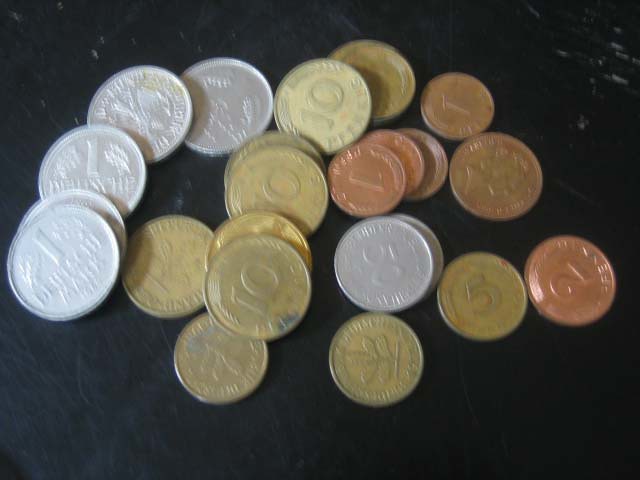This image shows a variety of scattered coins on a black surface table, which is notably scratched on the top right side, revealing a grayish layer beneath. The coins are arranged mostly from the left center, forming slight curves and overlapping in some places. Starting on the left, there are five silver coins marked with the number '1' and an inscription that reads "douche mark." Next to these, to the right, is a single gold-colored coin with the number '10' on it. Further to the right, there's a row of six gold coins, with three visibly marked '10' and the rest having unclear etchings. 

Above these gold coins and slightly to the right, there is a small copper coin with a '1' on it. Just below, there are three smaller copper coins stacked on each other, also marked with '1'. To the right of these, there's a larger copper coin, roughly the size of a quarter, featuring an etching of a woman's face. Down and to the left of this coin, two silver coins are stacked, each marked with '50' and surrounded by intricate etchings. Beneath these, there's a copper coin with a plant-like etching on it. Moving up and to the right, there is a copper coin marked with '5', and to its right, a darker copper coin with a '2' inscribed on it. The coins vary from silver and gold to different shades of copper, featuring various denominations and designs.